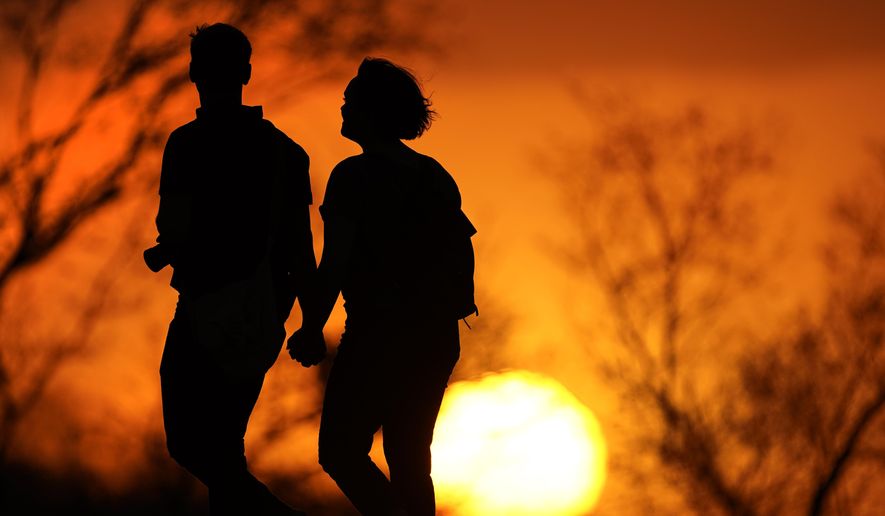In this evocative photograph captured at sunset, a couple, silhouetted against a sky ablaze with warm hues of yellow, gold, burnt orange, and umber, walk hand-in-hand towards the left. Their backs are turned to the photographer, their identities shrouded in shadows, enhancing the romantic mystery of the scene. The woman, with her short hair, and the man, possibly sporting a crew cut and what looks like a camera hanging around his neck, seem lost in the moment. They are surrounded by the stark, bare branches of leafless trees, suggesting a fall or winter setting, yet their light attire indicates mild weather. The sun, immense and golden, is just beginning to kiss the horizon, casting the entire scene in a serene, golden glow. The intricate network of tree branches in the background adds a textured depth, making the couple’s serene walk through this wooded area an intimate and timeless depiction of quiet togetherness.